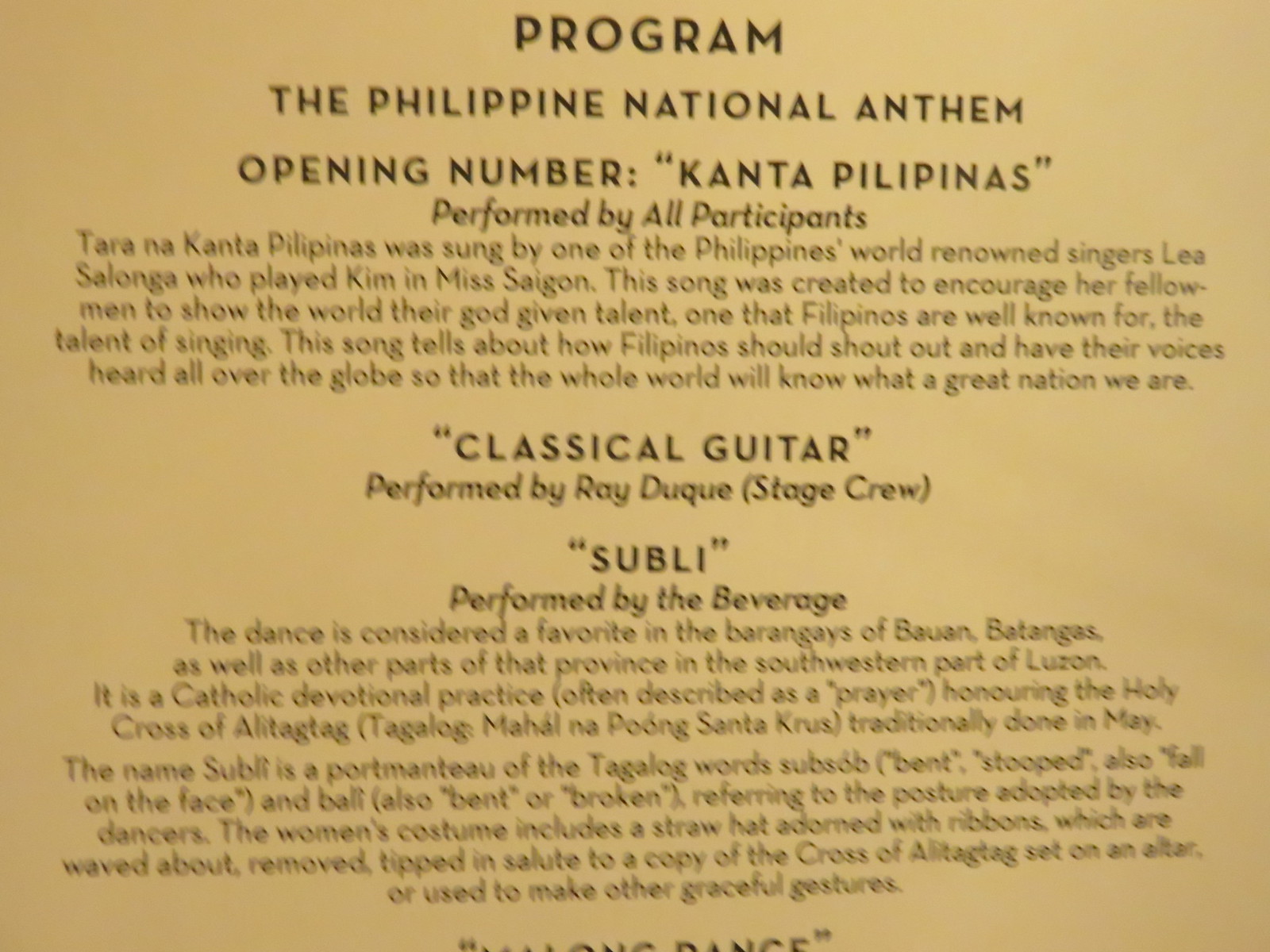The image depicts an old beige-colored program with slightly blurry black text, centered and neatly aligned. At the top, it prominently displays the word "PROGRAM," followed by a detailed listing of performances. The sequence begins with "The Philippine National Anthem," and the opening number, "Canta Filipinas," performed by all participants. This song, sung by Lea Salonga—an internationally acclaimed Philippine singer known for her role as Kim in "Miss Saigon"—was created to inspire Filipinos to showcase their exceptional singing talent to the world. The lyrics encourage Filipinos to proclaim their voices globally, celebrating their nation’s greatness. Following this, the program lists a "Classical Guitar" performance by Ray Duque of the stage crew. Next is "Subli," performed by The Beverage, described as a favored traditional dance in the barangays of Buwan, Batangas, and other regions in southwestern Luzon. This Catholic devotional dance, often performed in May, honors the Holy Cross of Alitagtag. The term "Subli" is a blend of Tagalog words denoting a bent or stooping posture, characteristic of the dance. The women's costumes include straw hats adorned with ribbons, which are waved, removed, or tipped in salute to a cross and used to make graceful gestures throughout the performance.